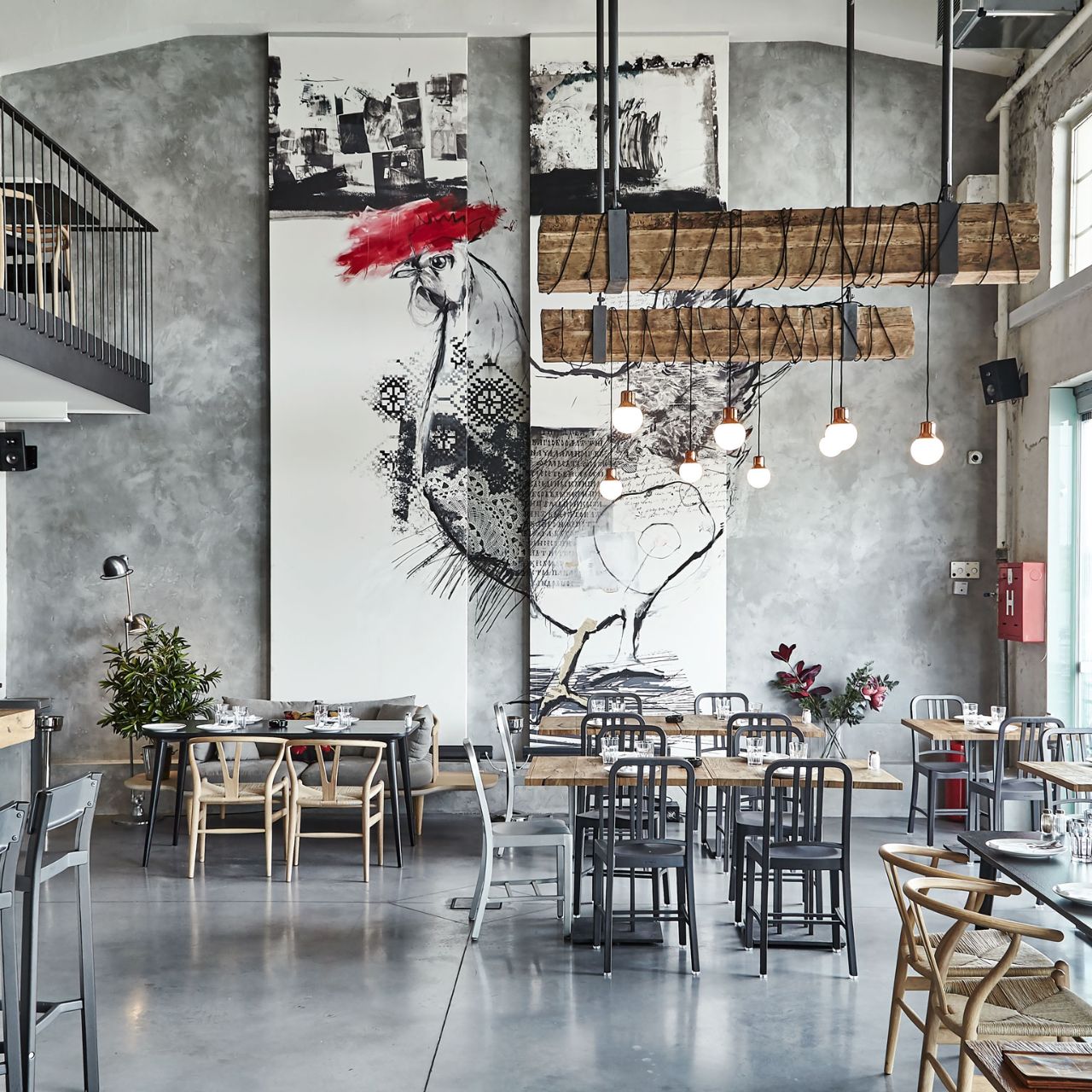The photograph captures a spacious, modern restaurant interior characterized by its polished concrete floor and plain gray concrete walls. Dominating the back wall, which appears to be about 20 feet high, is an eye-catching black and white mural of a chicken. This mural is spread across two white pillars that protrude slightly from the wall, with the chicken's head on the left pillar, its body in the middle, and its tail on the right. 

From the ceiling hang large brown wooden beams supported by black metal pieces, alongside light fixtures featuring exposed bulbs. Additionally, white globe lights add a soft glow to the well-lit, bright space. The upper left corner of the image reveals a balcony with black railings, giving a glimpse of a second story.

On the right side of the photograph, there are two windows, one above the other, allowing natural light to flood the room. The dining area on the ground level is populated with diverse seating arrangements: tables with black tops accompanied by brown wooden chairs, wooden tables flanked by black and silver chairs, and a counter on the left side with stools. Behind one of the tables at the rear, a couch adds a touch of comfort, while potted plants enhance the overall ambiance.